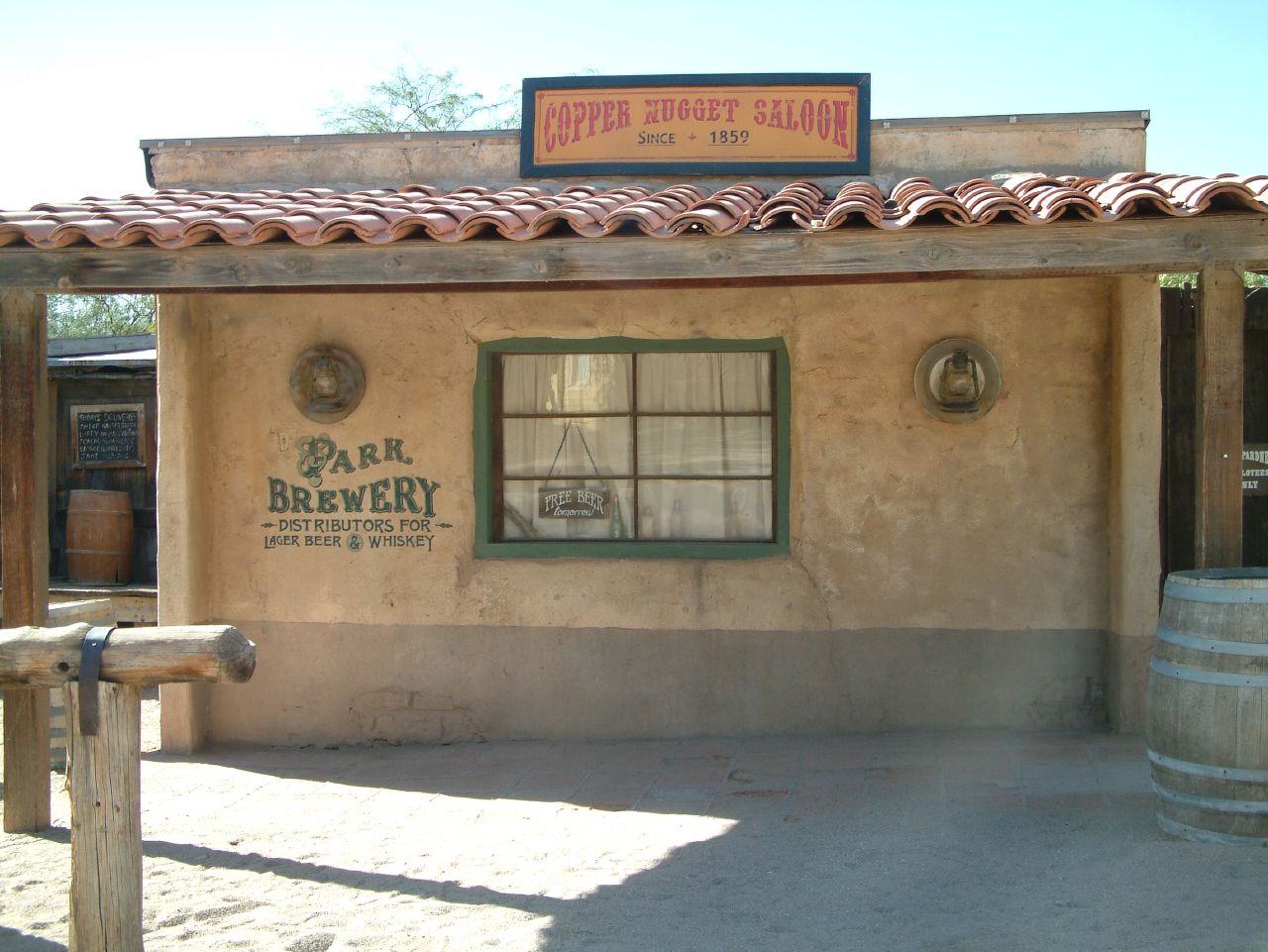This outdoor daytime photograph depicts the Copper Nugget Saloon, established in 1859, a single-story building with a terracotta roof made of curved shingles. The structure appears to be adobe with an old architectural style, featuring a single window with a green frame. A sign in the window promises "Free Beer," while painted on the wall next to it are the words "Park Brewery Distributors for Lager Beer Whiskey." A wooden hitching post stands prominently in the sand-covered foreground on the left side, suggesting a historical touch where patrons might have once tied their horses. To the right of the window, a wooden barrel with metal bands adds to the rustic charm. The background reveals a clear blue sky with a tree, completing this picturesque scene that harks back to the saloon's storied past.